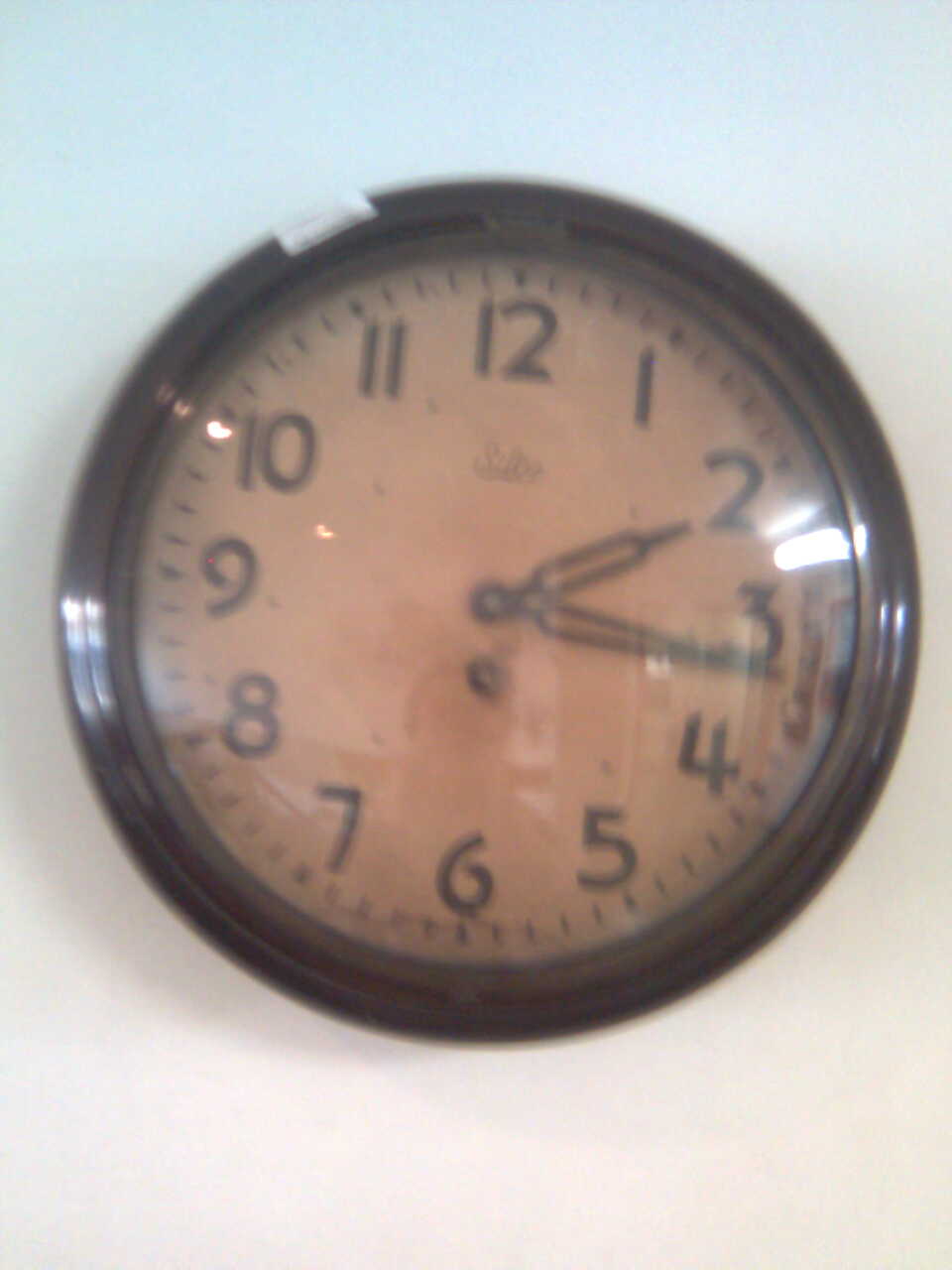This image depicts an old wall clock set against a white wall. The clock's housing appears to be a dark brown or black, with a reflective surface that casts shadows, including one of the photographer. The clock face is tan or brown, possibly due to aging, and encircled by a gray border. It features black numerals from 1 to 12, along with tick marks for minutes. The clock hands, designed in a decorative wire frame style, indicate the time to be around 2:17. Just below the 12, there is some script writing that is not clearly readable. The image is slightly blurry, possibly due to lighting reflections that add a gradient effect from light blue at the top to a pinkish hue at the bottom. There is also a small white mark near the top left of the clock frame.